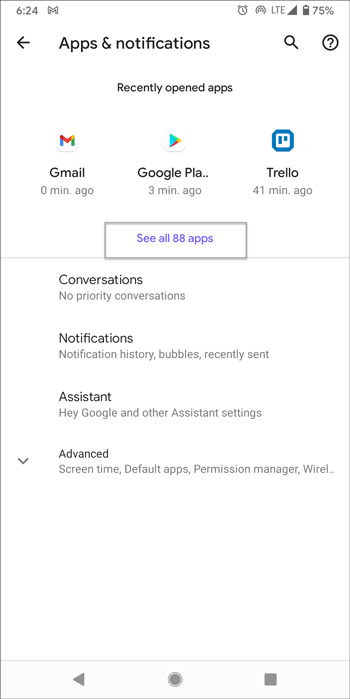Detailed Caption: 
In this color portrait-format screenshot from a smartphone taken at 6:24 AM, several on-screen details are visible. The top-left corner shows the time as 6:24, alongside the icons for Gmail and an alarm clock. The status bar indicates a full cellular connection and a 75% battery life. The main screen is displaying the "Apps & notifications" settings page. At the top, it lists "Recently opened apps," which include Gmail (opened 0 minutes ago), Google Play Store (opened 3 minutes ago), and Trello (opened 41 minutes ago). There is an option to "see all 88 apps" for a comprehensive list.

Beneath this section, several other settings categories are visible:
- **Conversations:** Displays "No priority conversations."
- **Notifications:** Options for "Notification history," "Bubbles," and "Recently sent."
- **Assistant:** Contains settings for "Hey Google" and other assistant features.
- **Advanced:** Includes options for "Screen time," "Default apps," "Permission manager," and more.

Each of these headings can be selected to access further detailed settings.